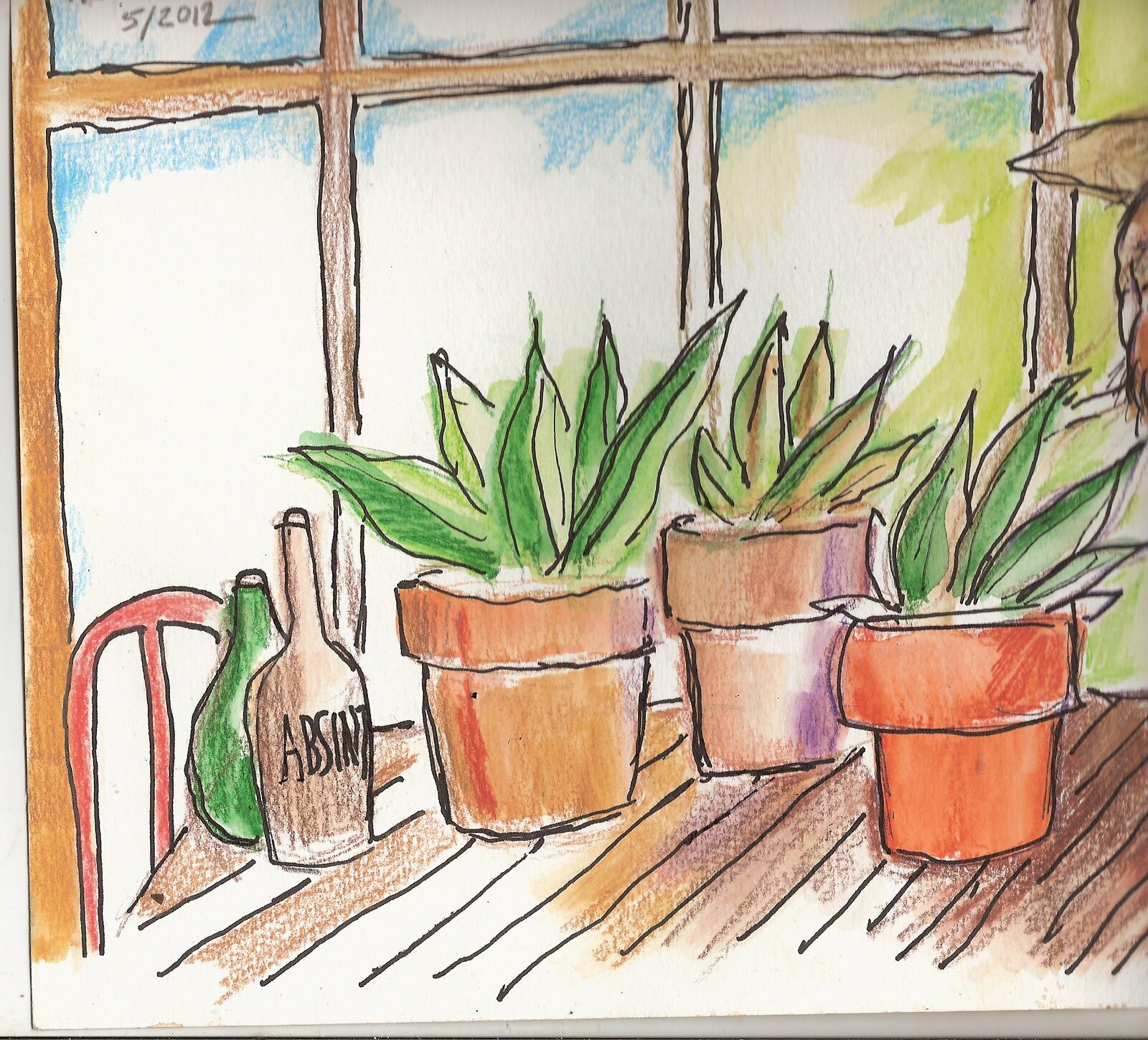This sketch, seemingly completed with pen and enhanced with crayon, captures a cozy, rustic scene featuring a wooden table with a vibrant red chair pulled up beside it. On the table, there are three potted aloe plants, each with four or five distinct green leaves jutting out of the pots. Next to the plants, two bottles are placed: one appears to be a brown liquor bottle, possibly of Absinthe, suggested by the partially visible label spelling "A-B-S-I-N-T", while the other is a green bottle of indeterminate content. The backdrop of the scene is a large window, providing a serene and welcoming ambiance to the overall composition.